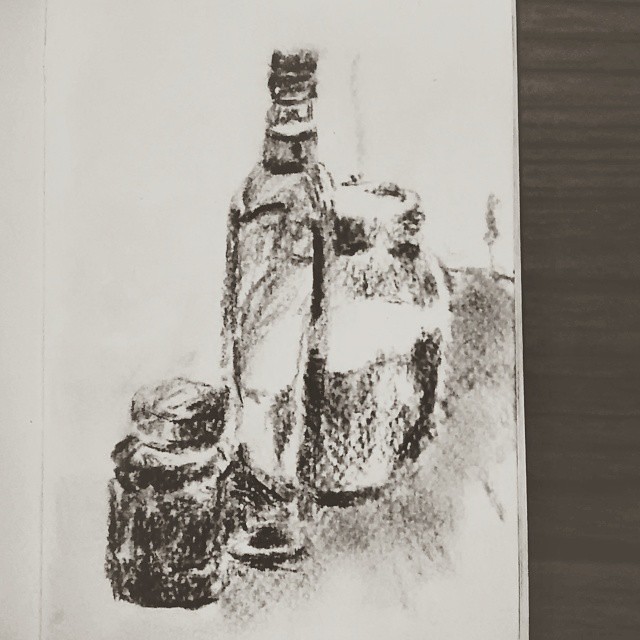This charcoal sketch, set against a contrasting black background, showcases a trio of objects meticulously rendered on white paper. Central to the composition is a tall bottle reminiscent of an olive oil container, capped with either a cork or screw top. To its right and slightly behind, a more rotund jar with a clearly defined screw top adds depth to the arrangement. In the foreground to the left of the tall bottle, a short, squatty bottle, heavily shaded to appear almost black, takes its place, resembling a salt shaker. Together, these elements create a harmonious still life study, with the artist's careful attention to detail and shading bringing texture and weight to the scene.